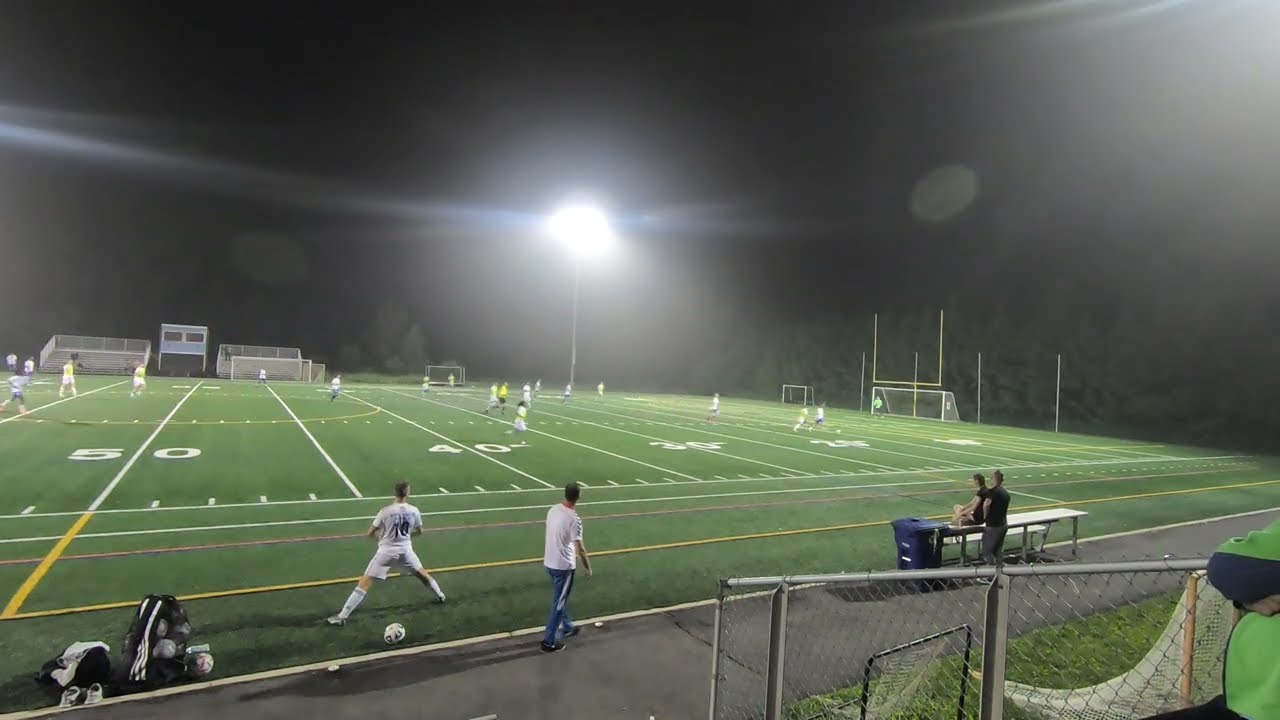This captivating night-time scene features a horizontally aligned rectangular image of a soccer game in progress on a football field. The dark, slightly blurry sky at the top contrasts with the brightly illuminated, clear green field below, marked with white yard lines for 50, 40, and 30 yards. The field, adapted for a soccer match, features visible goalposts on the right. Player activity is spread across the field, with players donning yellow and white jerseys. A long, gray walkway runs diagonally along the bottom left corner, where a white table hosts a woman seated and a man standing behind her. Near the bottom left, a soccer player in a white jersey with the number 10 and blue lettering stretches with a soccer ball and some gear nearby. Positioned on the lower right is part of a metal wire fence, adjacent to which a man believed to be the coach is walking, dressed in black or blue athletic pants and a white t-shirt. The image’s far horizon shows gray bleachers faintly visible, with a tall, bright, white lamppost illuminating the field. Additional features include a pink line along the edge of the field and yellow lines at the far edge. The scene is completed with two people interacting around a table near a tall blue trash can, all against the backdrop of a lively nighttime game.